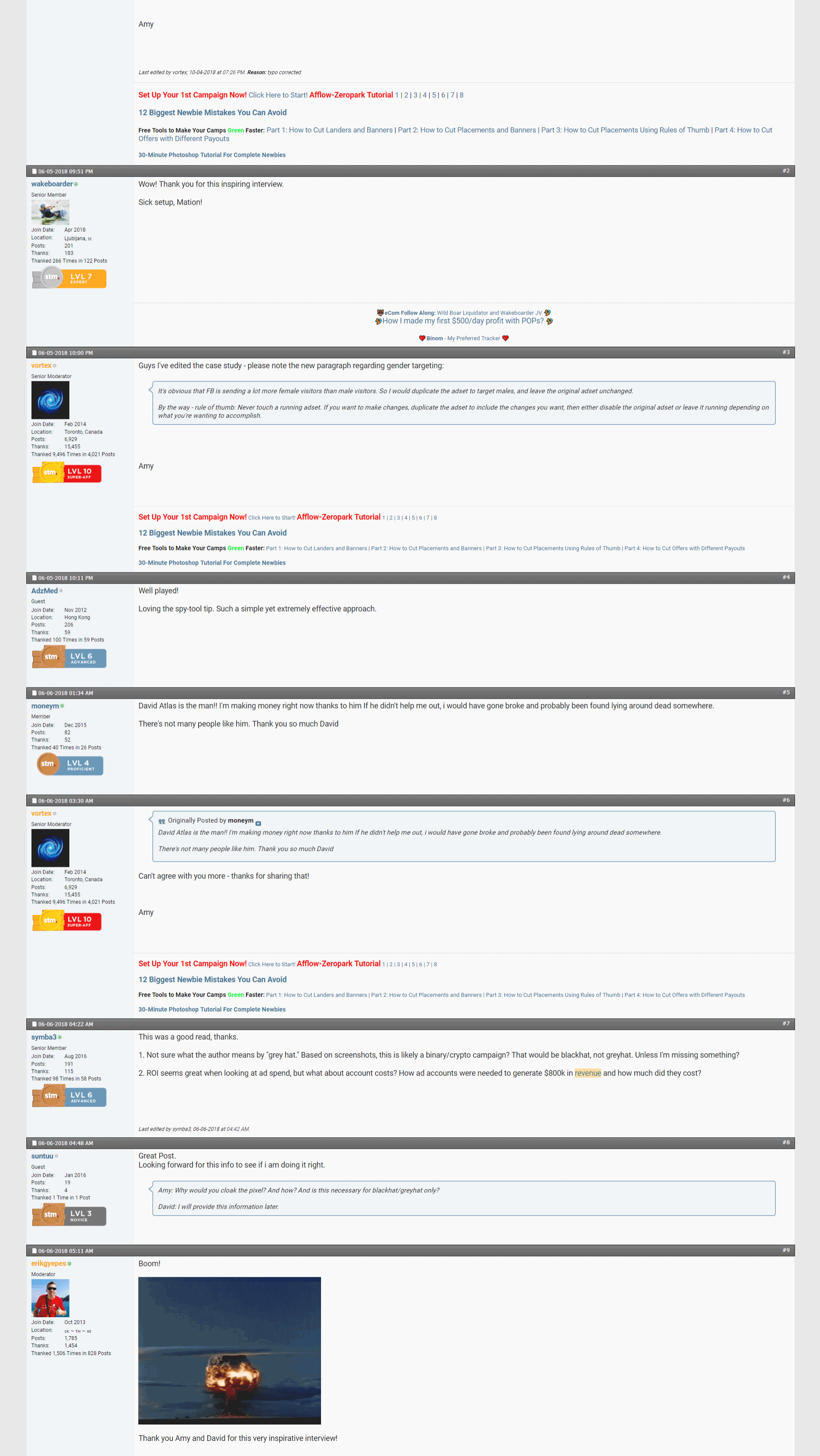A vertical screenshot captured from a smartphone or computer screen displays a detailed conversation forum. The sides of the image feature dark gray vertical strips, while the top and bottom remain unobstructed.

The forum is organized into several horizontal sections, each distinguished by a light bluish-gray vertical rectangle on the left side and a lighter gray rectangle spanning horizontally. At the boundaries of each section, a thin dark gray strip separates the entries.

At the top of the image, a message from Amy, highlighted in red, prompts, "Set up your first campaign now, click here to start." Below this introductory segment, multiple posts are arranged in chronological order.

Each post contains detailed user information: the date and time of the comment, the user's name, their profile picture, and additional personal details. Adjacent to this information, the user's message is displayed. 

For instance, one message reads, "Wow, thank you for this inspiring interview. Sick set up. - Matthew Machen." This pattern repeats throughout the forum, with various users participating, their names on the left, and their corresponding messages on the right.